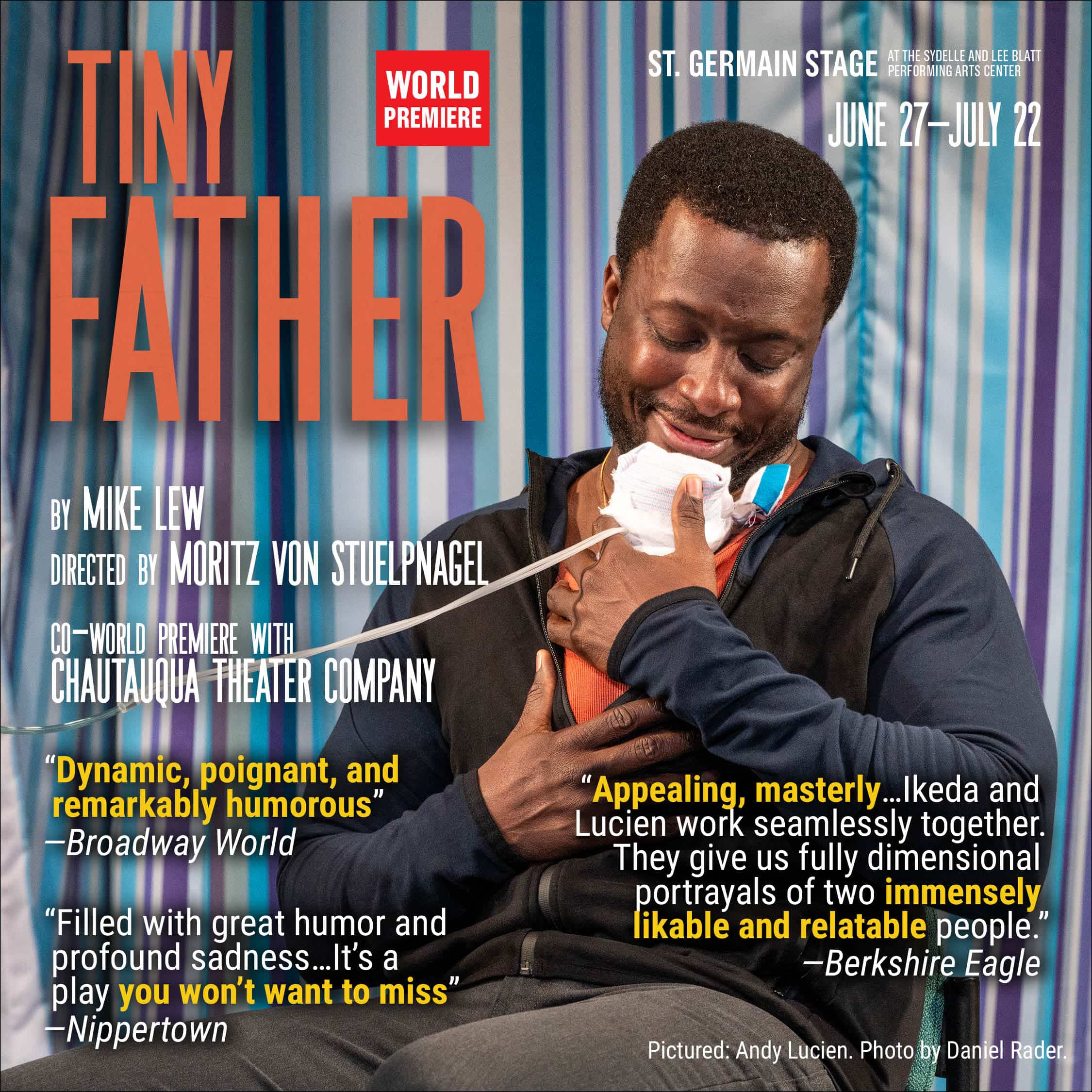Tiny Father: World Premiere

The poster for the event "Tiny Father" features an eye-catching design with the title written in a tall, thin, orange font located in the upper left corner. To the right of the title, a red rectangle with white text proudly announces "World Premiere." The event is scheduled to be held at the St. Germain Stage, part of the Sadella and Lee Blatt Performing Arts Center, running from June 27th to July 22nd.

Central to the poster is a poignant and touching image of an African-American man seated and holding a tiny baby—likely premature—close to his chest. The baby, whose head is covered and adorned with some kind of tubing, evokes a deep emotional response as the man looks down lovingly. The man is dressed in an orange t-shirt under a black and blue hoodie with gray pants, set against a backdrop of striped colors in hues of white, blue, purple, and light blue.

The poster also includes glowing reviews and credits, with quotes praising the show as "dynamic, poignant, and remarkably humorous" by Broadway World, and "filled with great humor and profound sadness," noted by Nippertown. Additional reviews highlight the show's emotional depth and relatable characters from the Berkshire Eco, praising the seamless work of Akita and Lucy. The play is written by Mike Liu and directed by Maritz van Stukenagel, with photography credits to Andy Lucey and Daniel Reiter.